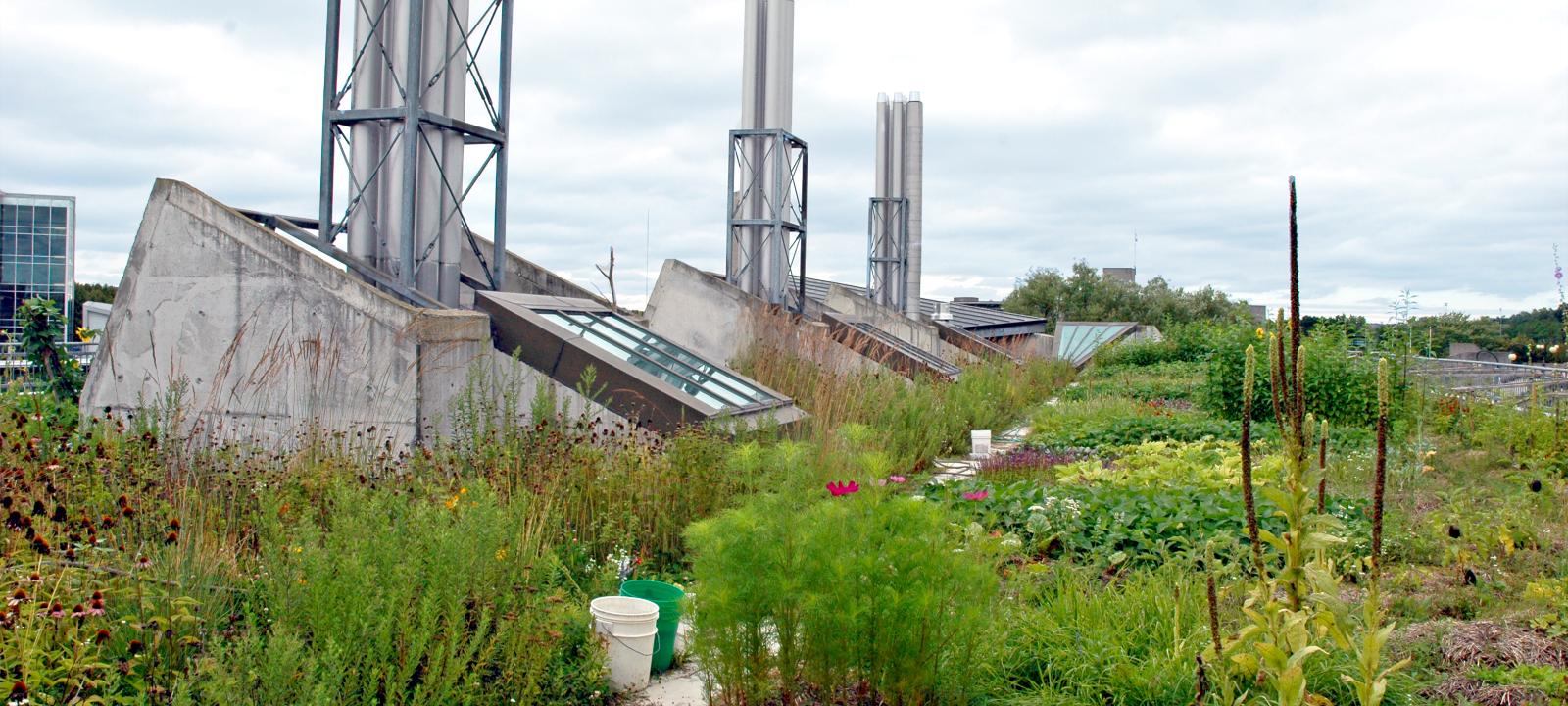This daylight photograph depicts an industrial site nestled in a verdant setting. Dominating the scene are three towering concrete structures, each reinforced with metal frame scaffolding at their bases, and arranged atop a slanted concrete foundation with windows that seem to provide light to the area below. Surrounding the industrial towers is a mix of overgrown grasses, various plants, and a few wildflowers adding specks of color to the greenery. Two buckets - one white, one green - are positioned on a path that winds through the plant life. In the background to the left, there stands a large four-story office building with an impressive glass facade, while another less detailed building with a glass front is visible as well, contrasting with the industrial elements in the foreground.